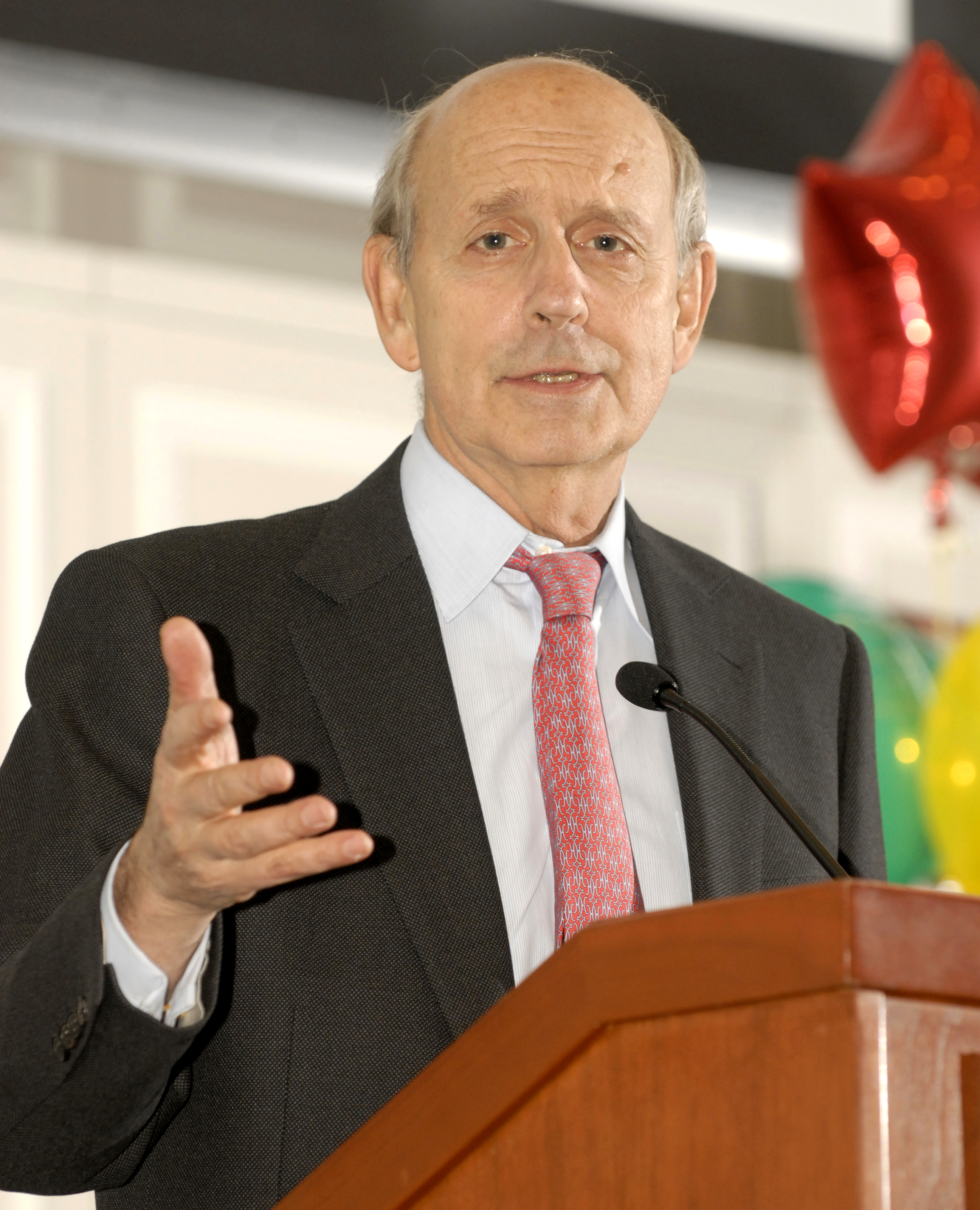This color photograph captures an older man standing behind a podium made of red-stained wood, situated in the bottom right corner of the image. The podium features a black microphone pointing toward the man's chest. The man, visible from the waist up, is dressed in a dark grey business coat with three buttons on the sleeve, a white button-up shirt, and a red necktie adorned with intricate grey and white patterns. His necktie is slightly loose, as he has not fastened the top button of his shirt. The man is bald on top with grey hair on the sides, and he faces forward toward the camera while his body is oriented to the right. He is gesturing with his right hand, palm open and facing to the right.

The man appears middle-aged to elderly, distinguished by light-colored eyes, an age spot on his forehead, and some wrinkles. Behind him, the backdrop consists of a white wall adorned with a partially visible green and yellow circular design. The festive setting is further accentuated by multiple balloons, including a reflective metallic red star and round balloons in green and yellow hues.